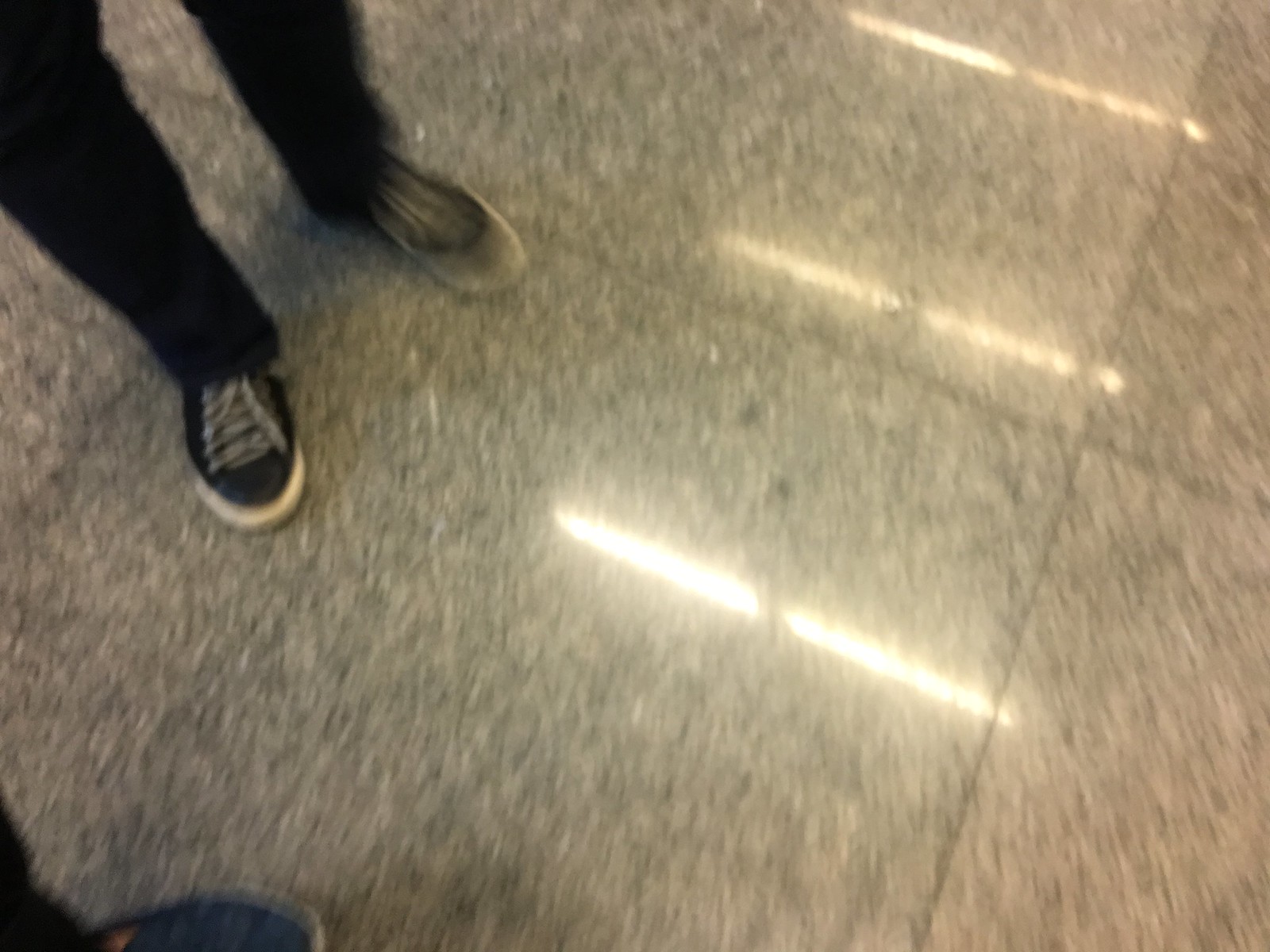The image captures an overhead view of a school hallway floor, composed of large, black and white checkered tiles that mimic the appearance of granite. In the top left corner, a person's legs are partially visible, dressed in black pants and black shoes with distinctive white soles. In the bottom left corner, a blue shoe with a white sole and part of a black pants leg come into view from the side. The floor reflects the ceiling's fluorescent light fixtures, with three sets of dual lights creating a pattern of bright spots towards the right side of the photograph.